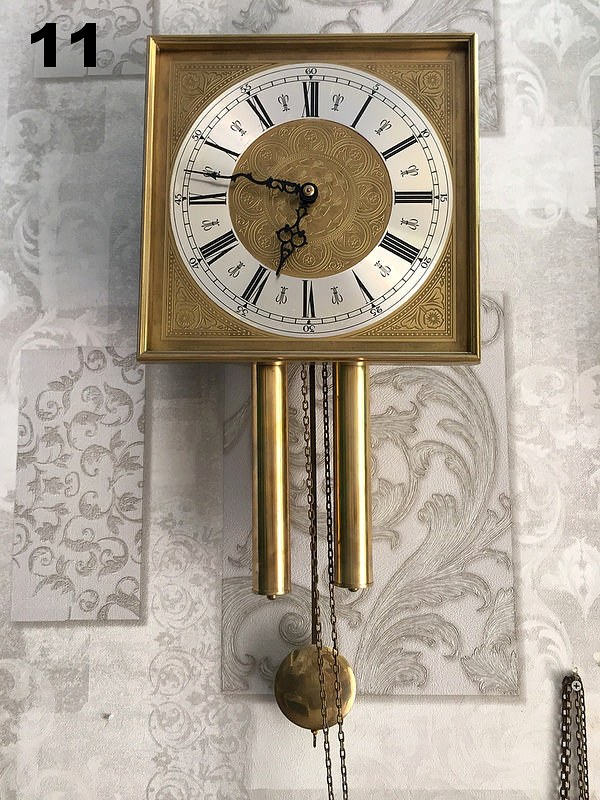The image depicts an opulent, brass-colored clock mounted on a wall adorned with highly ornate, silverish-gray wallpaper featuring intricate, abstract, floral or paisley patterns. The clock itself is square-shaped with a circular white dial showcasing Roman numerals and delicately crafted minute and hour hands. The dial is surrounded by detailed floral and dotted brass embellishments, both on the outer frame and the clock face. Below the clock face hang a brass pendulum and two matching weights, accompanied by a decorative chain extending downwards. The precise time indicated is approximately 6:47. In the upper left corner of the image, the number 11 is displayed in black font, suggesting an exhibition or sample unit designation. The overall aesthetic is lavish and meticulously detailed, making it hard to ascertain whether the setting is a private residence or a display environment.